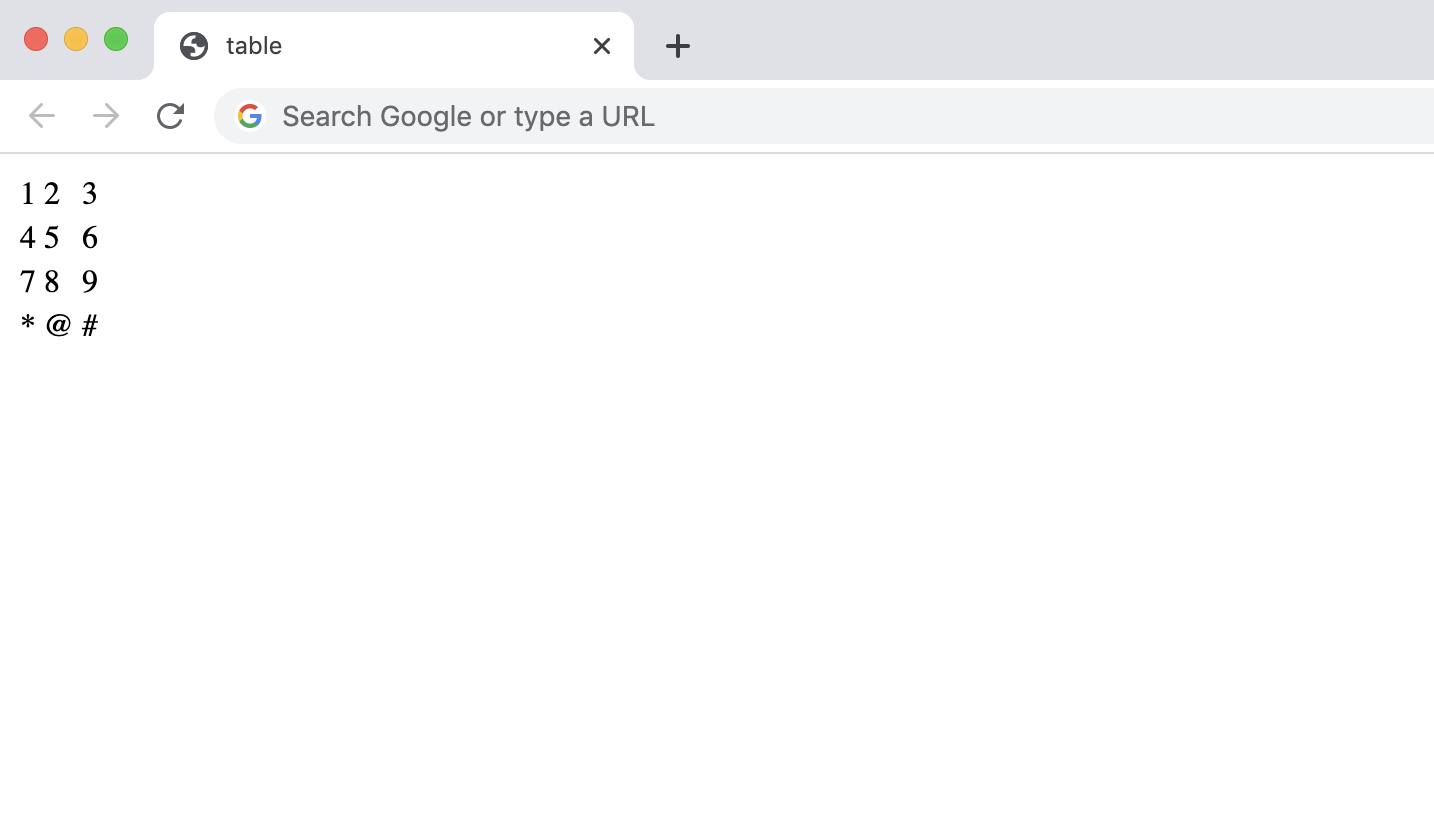A detailed screenshot of a computer screen showcases a series of features. On the far left, there are three solid-colored circles: a small red dot, a yellow dot, and a green dot arranged vertically. To the right of these dots, there is a tab labeled "Table" featuring a black and white globe icon, which indicates a browser environment. Adjacent to the tab label is an "X" icon for closing the tab, and a "+" icon for opening a new one. Further to the right, navigation arrows (left and right) are present, along with a refresh button. Below this navigation bar is a search or URL input field marked with the Google logo. The main content area displays a grid of numbers in black font, organized into rows. The first row consists of numbers 1, 2, and 3; the second row contains 4, 5, and 6; the third row features 7, 8, and 9; and the last row includes symbols: an asterisk (*), an at symbol (@), and a number symbol (#).